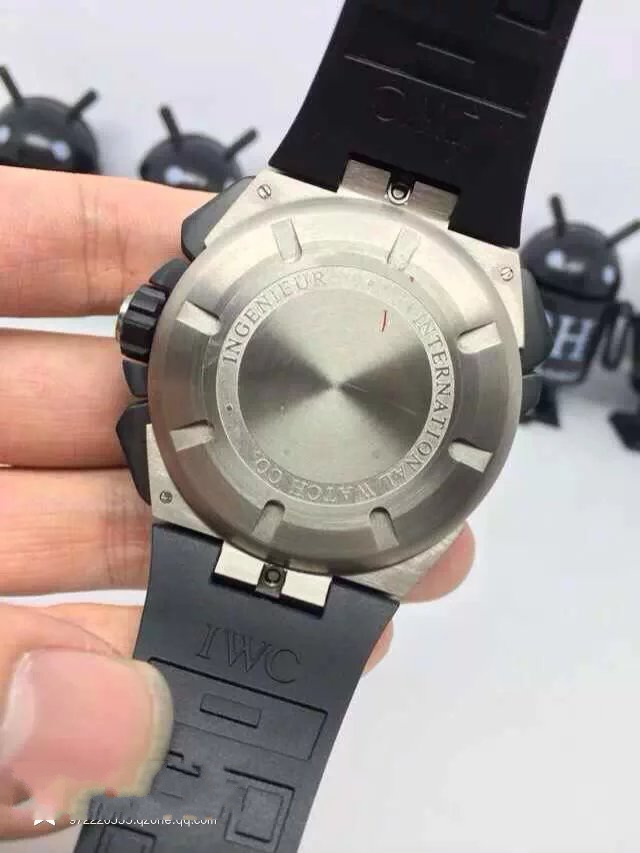This detailed photograph, taken against a solid white background, appears to be captured inside a store. It prominently features a close-up view of a watch held by a left hand, with visible nails and fingers. The watch is a product of the International Watch Company (IWC), branded as Ingenieur. The watch has a black rubber wristband, contrasting with its gleaming silver chrome back plating. Inscribed on the back are the words "Ingenieur International Watch Company" in a cylindrical pattern. The watch is of the flip-top variety, and in the photo, its cover is closed, obscuring the face. Adding to the intricate design, the watch features a black stem with a silver tip and slight U-shaped notches on its outer edge.

In the blurred background, rows of robot toys can be discerned, characterized by their black cylindrical bodies marked with a white letter "H," black square bases, black arms, and black dome heads with antennae. These robots also have distinctive, wide triangular white eyes. The overall composition of the image is focused on the watch in the foreground, with the white backdrop providing a stark contrast enhancing the scene's details and clarity.